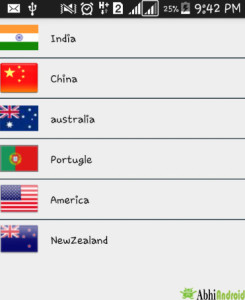The image depicts a cell phone screen with several indicators and flags:

- At the top left, there is an envelope icon indicating the presence of new mail.
- Next to it, an alarm icon shows the sound is turned off.
- The signal bars for the phone display a current network connection, and the battery icon indicates a 25% charge at 9:42 PM.

Below these indicators, there is a series of flags each separated by black lines:
1. The first flag features stripes of orange, white, and green, representing India.
2. The second flag shows five yellow stars on a red background, symbolizing China.
3. The third flag has the Union Jack in the upper left corner on a blue field with white stars, representing Australia.
4. The fourth flag is green and red with an emblem in the center, signifying Portugal.
5. The fifth flag is white and blue with stars, representing the United States.
6. The sixth flag has the Union Jack in the upper left corner and blue stars on a blue field, representing New Zealand.

In the bottom right corner, there's text reading "Il a BHI Android," displayed in black and green, accompanied by a small Android mascot. The top band of the screen is black with white icons, and all the colors are present in the flags.